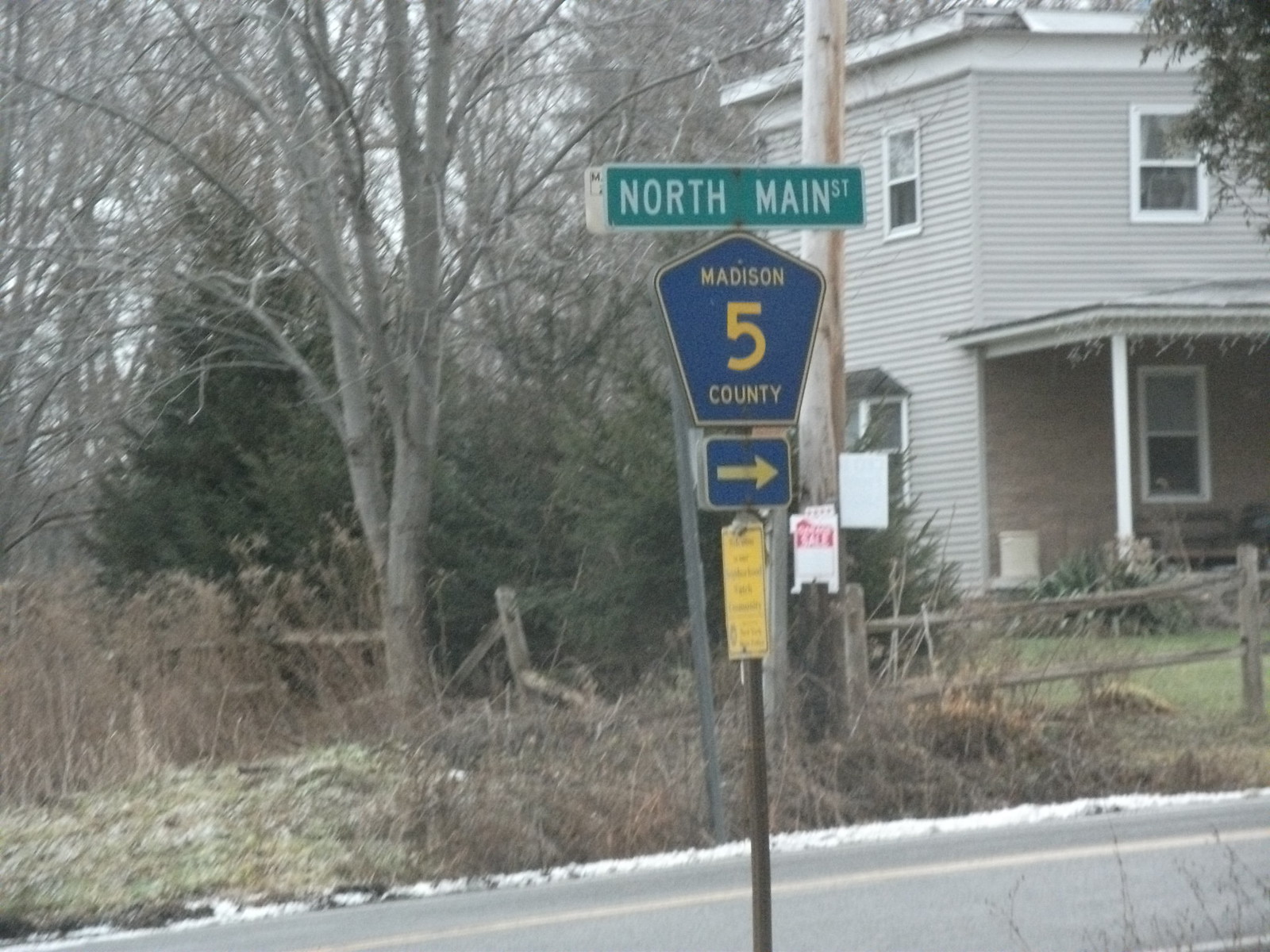In this photograph, we see an up-close view of a street sign situated in the middle of a street, adjacent to a large two-story house. The street sign prominently features "North Main Street" at the top, with a green background and bold white lettering. Just below, there is a blue sign indicating "Madison 5 County," displayed within a five-sided symbol reminiscent of a stop sign, though slightly different. Below that is a blue sign with a yellow right arrow, directing towards Madison 5 County. The wooden pole holding these signs is brown, extending into a street marked by a double yellow line.

To the right of the image, the two-story house is notable with its white horizontal siding and white trim around transparent windows. The house also boasts a small patio supported by a white pillar and has icicle Christmas lights adorning the front porch, though they are unlit as it is daytime. The roof appears flat, which is somewhat unusual. The surrounding landscape includes a broken-down fence, an old dead tree to the left, a mix of green plants, dead grass, and patches of snow along the curb. The overall atmosphere evokes a winter day, characterized by a gray and overcast sky, devoid of sunlight.